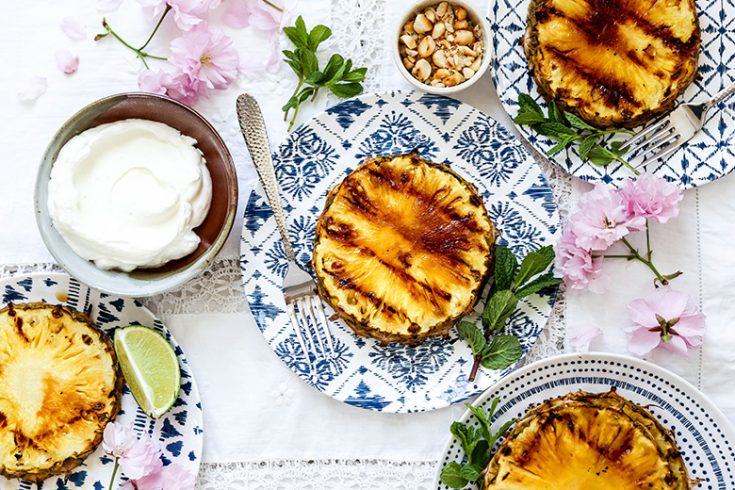The image showcases a charming display of various foods arranged on different blue-and-white plates with intricate patterns. Each plate features at least one piece of round, char-marked, grilled pineapple, accompanied by vibrant green sprigs as garnish. The plates sit atop a white lacy tablecloth and are surrounded by delicate pink flowers, enhancing the visual appeal. In addition to the pineapple, there is a bowl filled with fluffy white whipped cream, positioned on the left side of the image. Other notable elements include a small cup containing chopped nuts, either peanuts, cashews, or possibly mushrooms, and a slice of lime on one of the plates. The meticulous arrangement and the colorful presentation make it an enticing and visually delightful display of grilled pineapple and accompaniments.